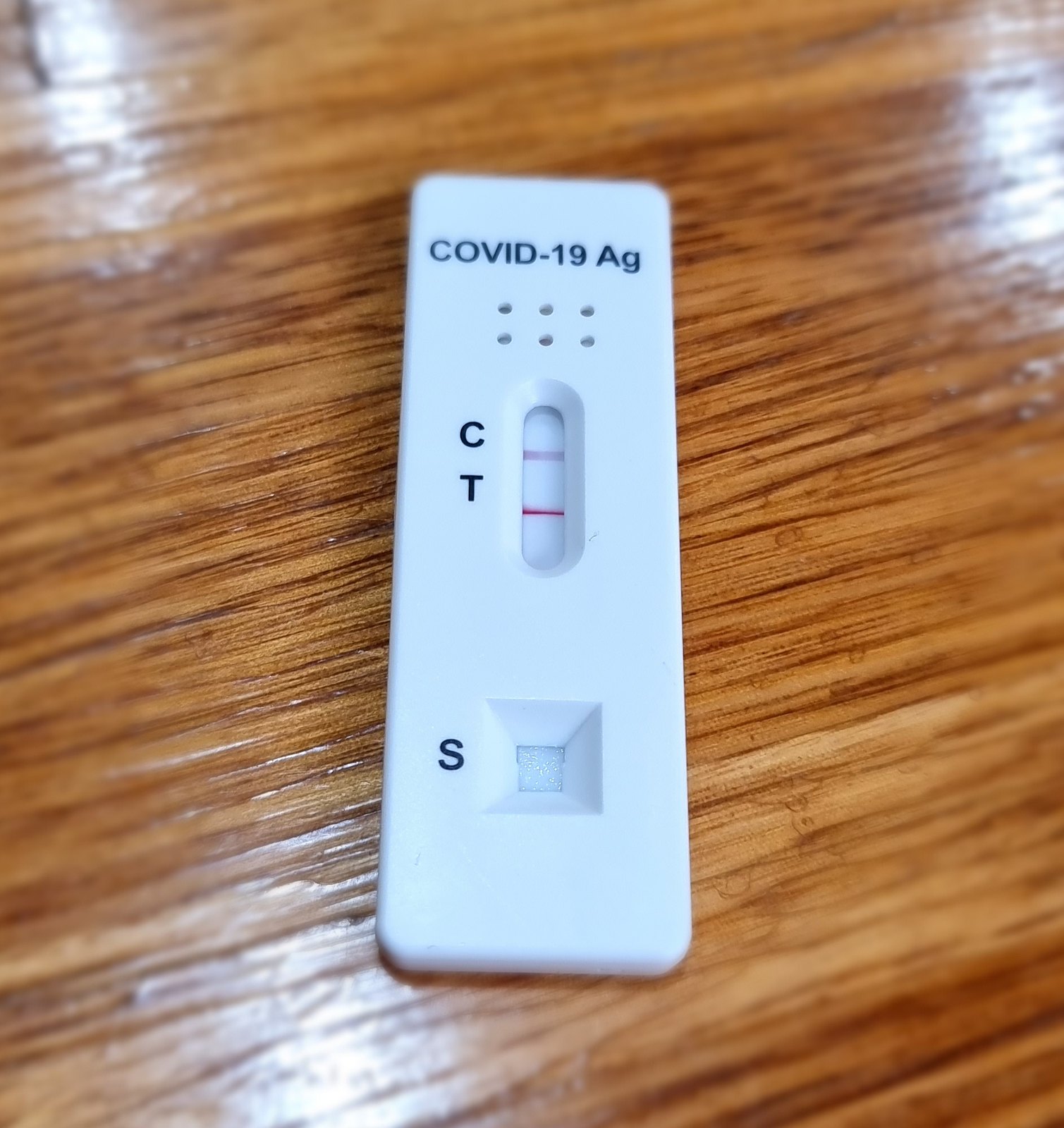This color photograph showcases a beautifully polished table surface made of medium to dark brown wood. The rich wood grain is accentuated by light reflections in the upper left corner, upper right corner, and along the bottom edge of the image.

Prominently displayed on the table is a single object: an elongated, white device. At the very top, it bears the label "COVID-19 AG" in bold block letters. Below this label are six small, evenly spaced holes arranged in two rows of three. Further down, the device features an oval-shaped window insert, within which is a single red line. Adjacent to this window, the letters "C" and "T" are vertically aligned, with "T" situated below "C". At the very bottom of the device is a small, cut-out square, empty and white, situated to the right of the letter "S" printed on the left side.